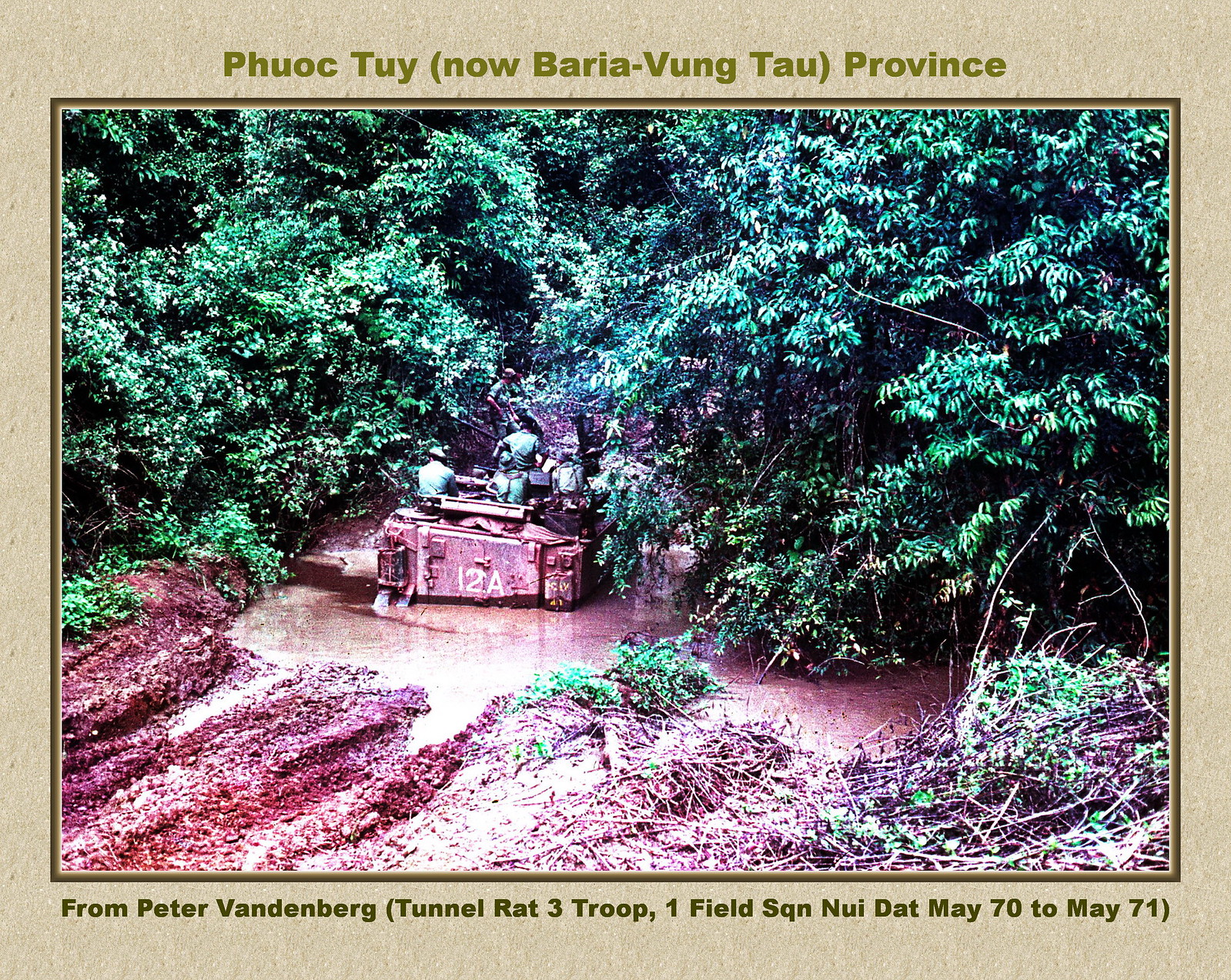This historical military photograph, bordered in tan brown, captures a scene from the Phuoc Tuy province—now known as Ba Ria-Vung Tau province—during the Vietnam War, dated between May 1970 and May 1971. The image features a group of four men clad in green military uniforms, standing in a flooded, muddy area surrounded by dense jungle foliage. Central to the scene is a half-track military vehicle partially submerged in water, identifiable by the metal structure it rests on, marked with "one, two, a". In the upper part of the vehicle, one soldier is visible, with his head sticking out. The foreground depicts a mix of reddish dirt, green shrubbery, and twigs. The top border captions "P-H-U-O-C-T-U-Y now Ba Ria-Vung Tau province," while the bottom border credits the photograph to Peter Vandenberg, identified as Tunnel Rat 3 Troop, 1 Field Squadron. This evocative image serves as a poignant reminder of the challenging conditions faced by soldiers during this period.